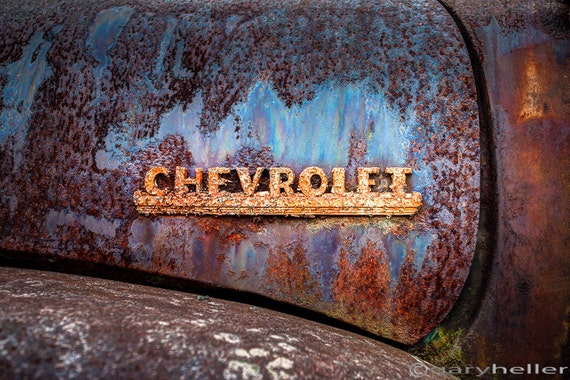This is a close-up photograph of a very old, vintage Chevrolet truck, focusing on the rusty and patinaed surface. The image captures the front fender and side portion of the hood, showcasing a fascinating blend of colors and textures. The original blue paint peeks through a layer of rusty red, creating an almost oily rainbow effect where the patina has developed. The centerpiece of the photograph is the rusted Chevrolet badge, in a light yellowish-gold hue, with each letter connected by a horizontal line at the bottom. The metal surface around the logo is heavily corroded, adding to the vintage charm. The photograph bears the copyright of Gary Heller in the bottom right corner.